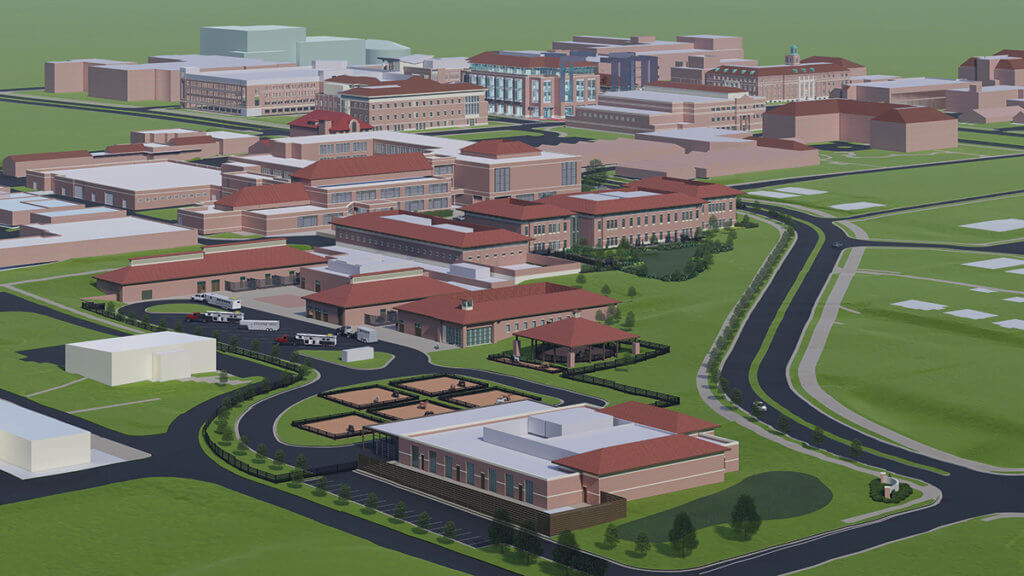This image is a 3D rendering of a city or large campus reminiscent of an early version of SimCity. The scene is dominated by organized, formulaic architecture with multiple buildings featuring windows and doors, many of which have brown exteriors with darker brown roofs, and a few distinguished by their pure white color. There are extensive green spaces, primarily grass fields interspersed with minimal tree coverage, and an intricate network of connecting roads and pathways that weave throughout the campus. A main road with white lanes curves around a central building that resembles a school, identifiable by its numerous doors. A solitary silver car is visible driving along this road. The entire layout, including parking lots with cars and a park-like area with brown lots, creates a cohesive system that underscores the interconnectedness of the site's elements. Despite the low detail rendering, the campus-like setting is clear, featuring notable buildings and minimal extraneous details, emphasizing a structured, almost simplistic cityscape.